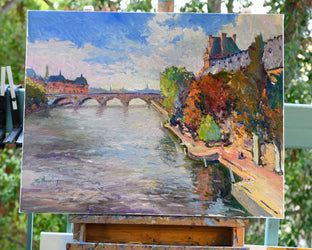The image is a photograph capturing an outdoor scene which features a painting. The setting includes a white wood fence with railings and large trees in the background. The painting, placed on an easel, nearly square in shape, depicts a serene river scene. The river, reflecting the colors of the sky and surrounding buildings, flows under a white stone arch bridge with a railing. To the left, there's a notable red-roofed structure possibly three or four stories high, and in the distance, a larger dome-like building is visible. The right side shows a light tan platform or dock adorned with vibrantly colored trees in hues of green, red, yellow, and slight blue. Streetlights are faintly discernible, and the sky in both the painting and the actual setting is dotted with clouds. The overall scene evokes a peaceful riverside ambiance, possibly reminiscent of Paris.